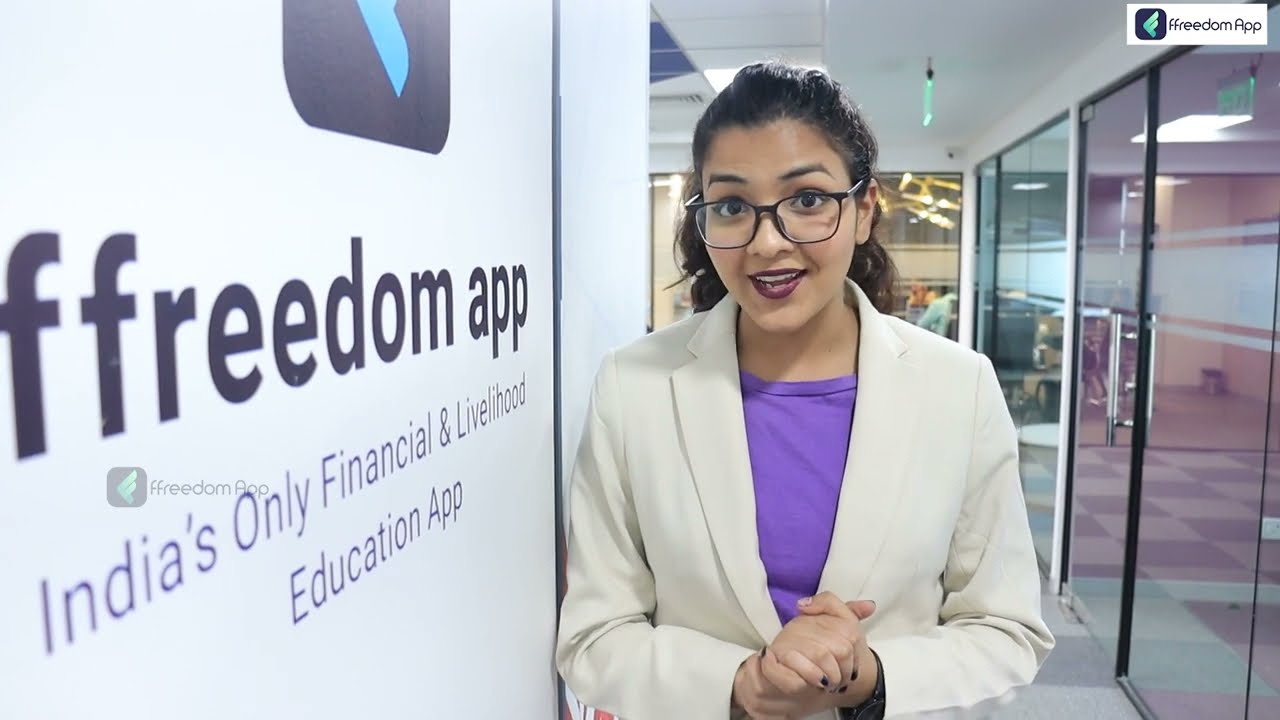The image, likely a screenshot from a promotional video, features a woman with darker skin and black hair pulled back in a ponytail. She is wearing black-framed glasses, a beige suit coat over a blue t-shirt, and has black nail polish. Her mouth is slightly open as if she is mid-sentence, and she is looking directly at the camera with her body facing forward, positioned slightly to the right of the center of the frame. Her hands are clasped together in front of her. 

She appears to be in an office setting, indicated by white and glass walls, and a nearby glass door. To her left, there is a white wall featuring signage that reads, "F Freedom App. India's only financial and livelihood education app," with the logo—a green, left-tilted "F" inside a black box—partially visible in the top right corner of the frame. The woman, possibly an ambassador for the app, seems to be explaining or discussing the app, adding a dynamic, engaged element to the composition.